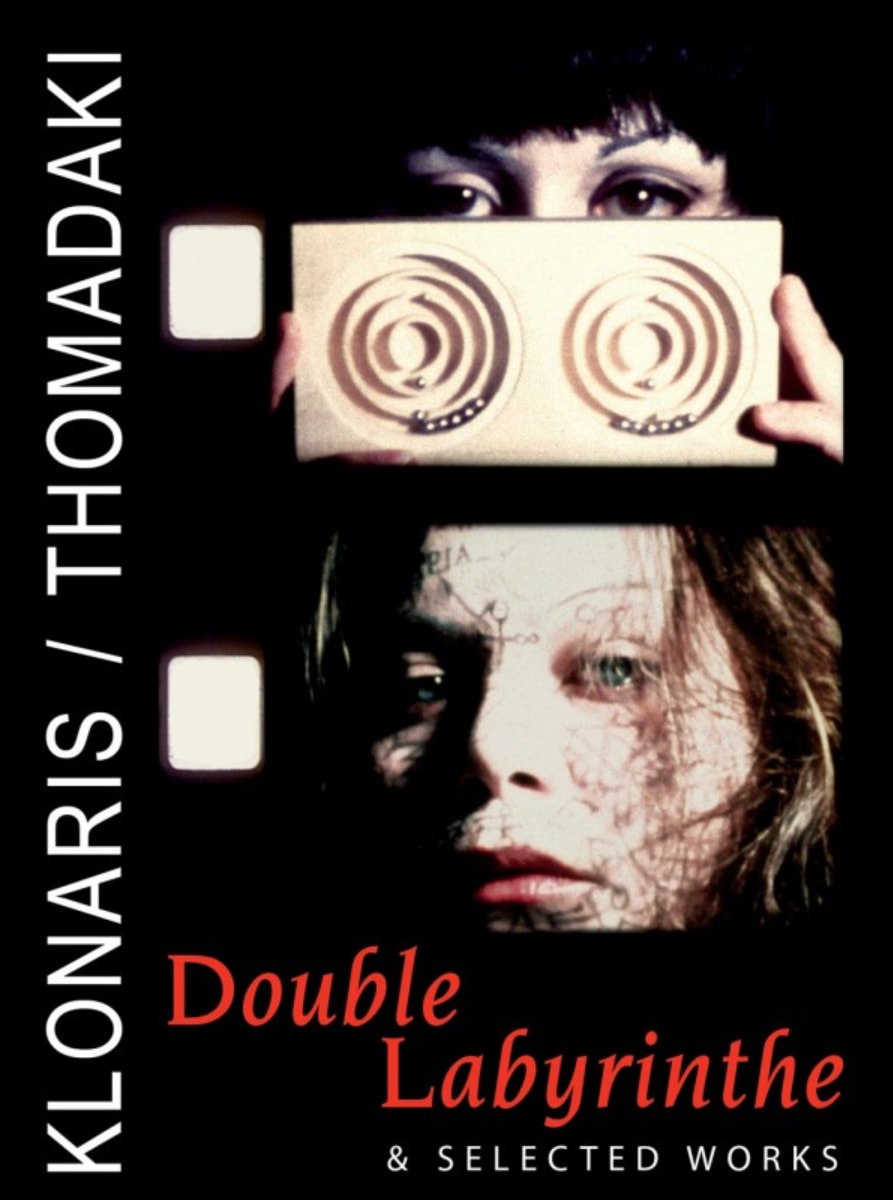The image is a detailed cover of a book, predominantly utilizing a black background. It features two stacked photographic portraits of women on the right side. The top photograph depicts a woman with elaborately made-up eyes, partially obscured by a handheld wooden game featuring concentric spirals designed as a labyrinth with silver balls aimed to reach the center. This woman's dark bangs cover her eyebrows, and her eyes are intently gazing at the viewer.

Below this, the second photograph shows a distressed woman with light blue eyes, light brown hair, and wisps hanging across her face. Her lips are slightly colored in a pale red, contrasting with the otherwise black-and-white palette of both photographs. This second woman also faces the viewer, but at a slight angle.

The left side of the cover displays bold white text rotated 90 degrees, reading "KLONARIS / THOMADAKI," suggesting the names of the authors or artists. At the bottom of the photographs, a red italicized text reads "Double Labyrinth," followed by smaller white text stating "& Selected Works."

Overall, the design cleverly integrates representationalism and realism through photographic and typographic elements, emphasizing the dramatic and haunting quality of the women's portraits against the stark black background.